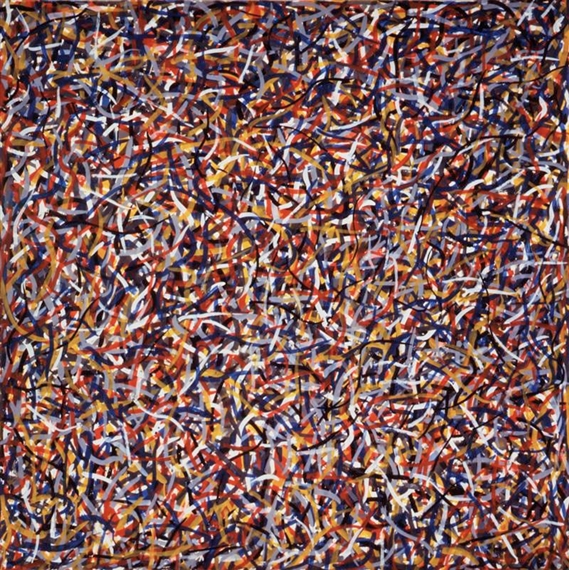The image is an abstract painting featuring a chaotic, dense assortment of thin, string-like ribbons and thread-like filaments, intertwined and evenly distributed throughout a large square frame. The vibrant color palette includes red, blue, green, yellow, orange, black, white, and even light blue. These colors are presented in various sections across the image and are bunched together so tightly that no background is visible. Vastly resembling a close-up photograph of scattered confetti, the ribbons range around a quarter of an inch in width, with black lines appearing thinner and more thread-like, often curving and bending like delicate eyebrows or wave-like shapes, adding a sense of dynamic motion to the composition. Despite the detailed individual strands, the image as a whole presents an impression of chaos and complexity, with no discernible objects, pictures, or text – just a mesmerizing interplay of colors and shapes.